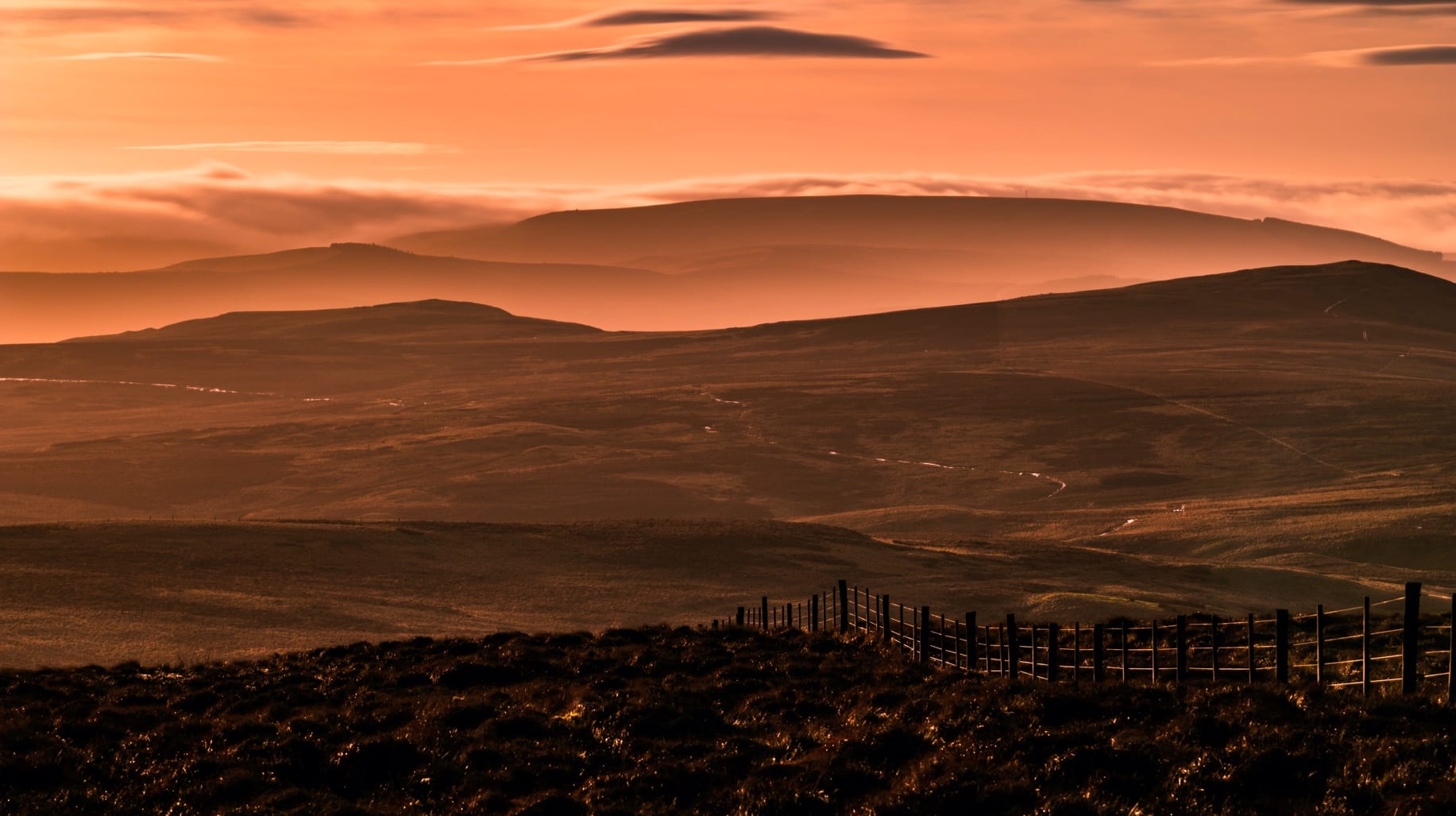This photograph depicts a striking landscape taken from an elevated vantage point, featuring a foreground dominated by darker colored grass, bushes, and a ground area covered with wet, black stones. In the lower right corner, a wooden and wire fence extends toward the middle of the image, delineating a vast, uneven field that transitions into rolling tan, black, and orange hills. A thin road meanders through these hills from the center to the middle left of the frame. Behind the hills, the scenery rises into a higher mountain framed against a dusky orange sky with a mix of white and dark gray clouds, enhanced by the warm, brownish-orange hues of a setting or rising sun. The entire scene exudes the serene, expansive beauty of ranch land under a captivating sky.